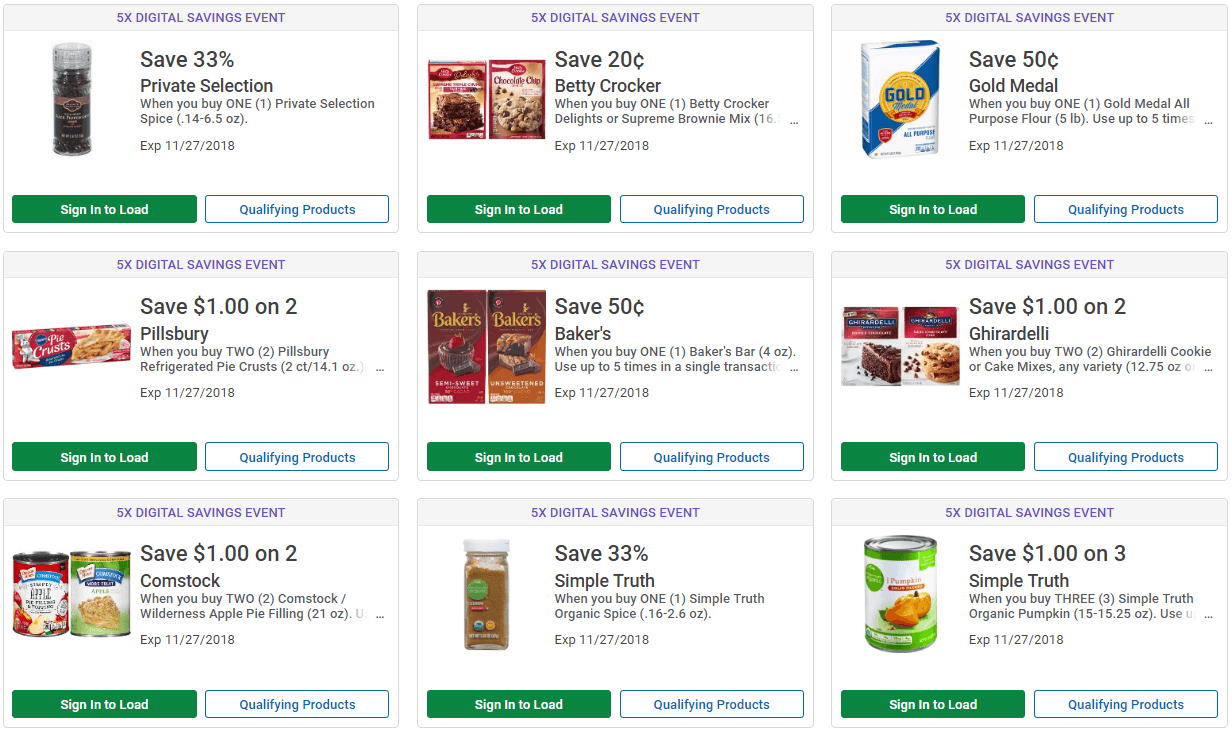The image features a selection of nine items available for sale on a website, presumably affiliated with Kroger, as indicated by the promotional banners and product brands. The top of the image displays a banner reading "5x Digital Savings Event: Save 33%" with a note specifically mentioning "Private Selection" spices as part of the deal.

To the right, there are various call-to-action buttons, including a green button labeled "Sign in to load" and another indicating "Qualified products," suggesting that the viewer needs to sign in to the website to activate or view these deals.

Each item in the grid comes with specific promotional details:

1. **Top Left:** Save $1.00 when you purchase two Fieldberry refrigerated pie crusts (2-count, 14.1 oz). The offer expires on November 27, 2018.
2. **Middle Left:** Save $1.00 when you purchase two Comstock Wilderness apple pie fillings (21 oz). The offer expires on November 27, 2018.
3. **Top Middle:** Save $0.20 on Betty Crocker when you buy one Betty Crocker Delights Supreme brownie mix. This offer also expires on November 27, 2018.

Additional items in the grid likely offer similar savings on various products, contributing to the overall promotional theme of significant savings during this digital event.

The visual arrangement and detailed text of the promotions are geared towards enticing customers to sign in and take advantage of these limited-time discounts on popular grocery items.